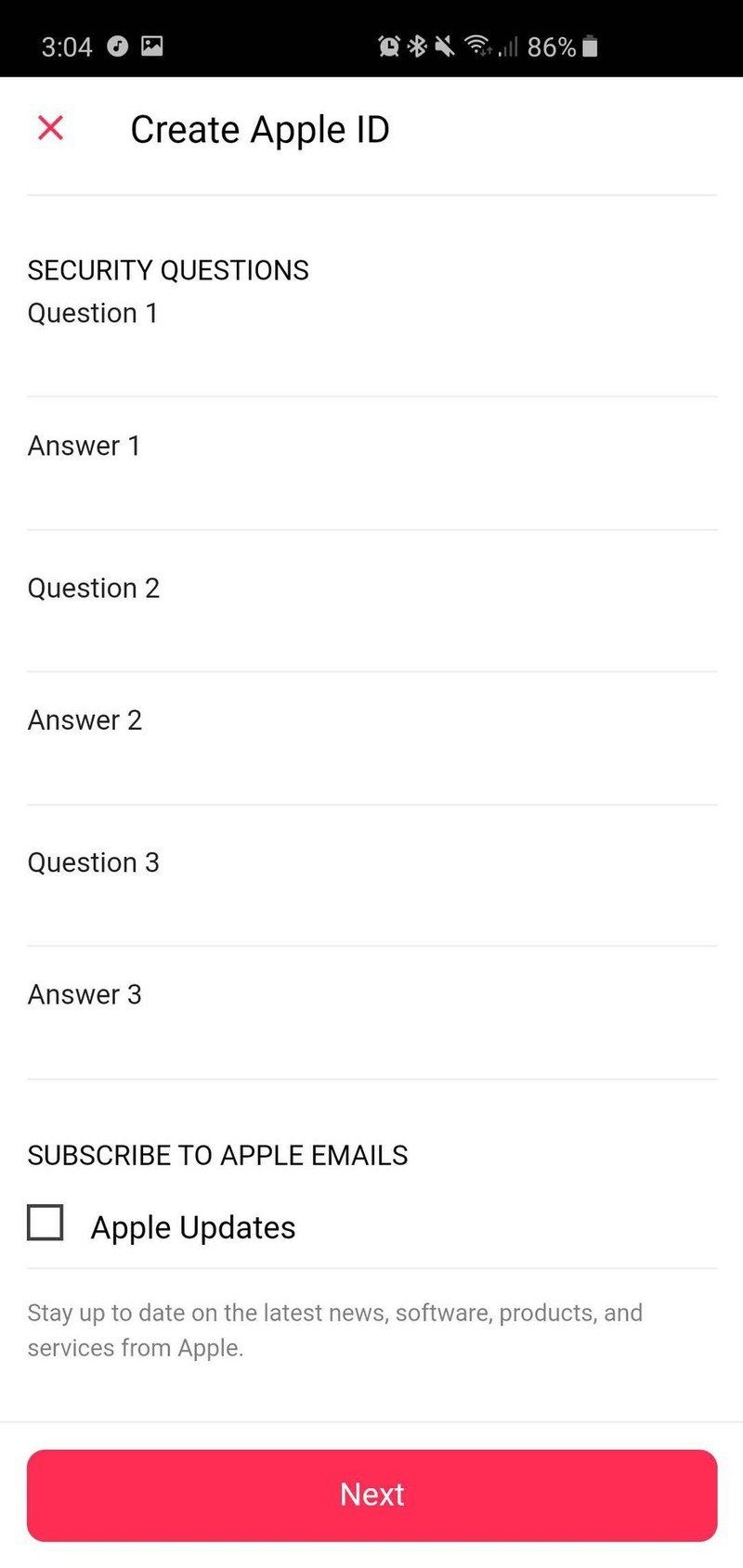Screenshot of a smartphone screen displaying the Apple ID creation page. The device clock reads 3:04 AM/PM at the top right corner, flanked by several status icons including an alarm clock, Bluetooth, volume control, Wi-Fi, and a battery level indicator at 86 percent. Below this status bar is the Apple ID creation interface starting with a red "X" button, followed by black text prompting the user to "Create Apple ID."

The screen shows fields for security questions, labeled "Question 1," "Answer 1," "Question 2," "Answer 2," and "Question 3," "Answer 3," respectively. Beneath these fields is an option to subscribe to Apple emails, indicated by an empty checkbox next to the text "Subscribe to Apple emails." The section elaborates with the sentence "Stay up to date on the latest news, software, products, and services from Apple."

The bottom section features a prominent red rectangle button, with the word "Next" in white centered within it. This image is a vertically-oriented screenshot without any photographic elements, people, animals, vehicles, or natural scenery, focusing entirely on the text and digital interface elements.